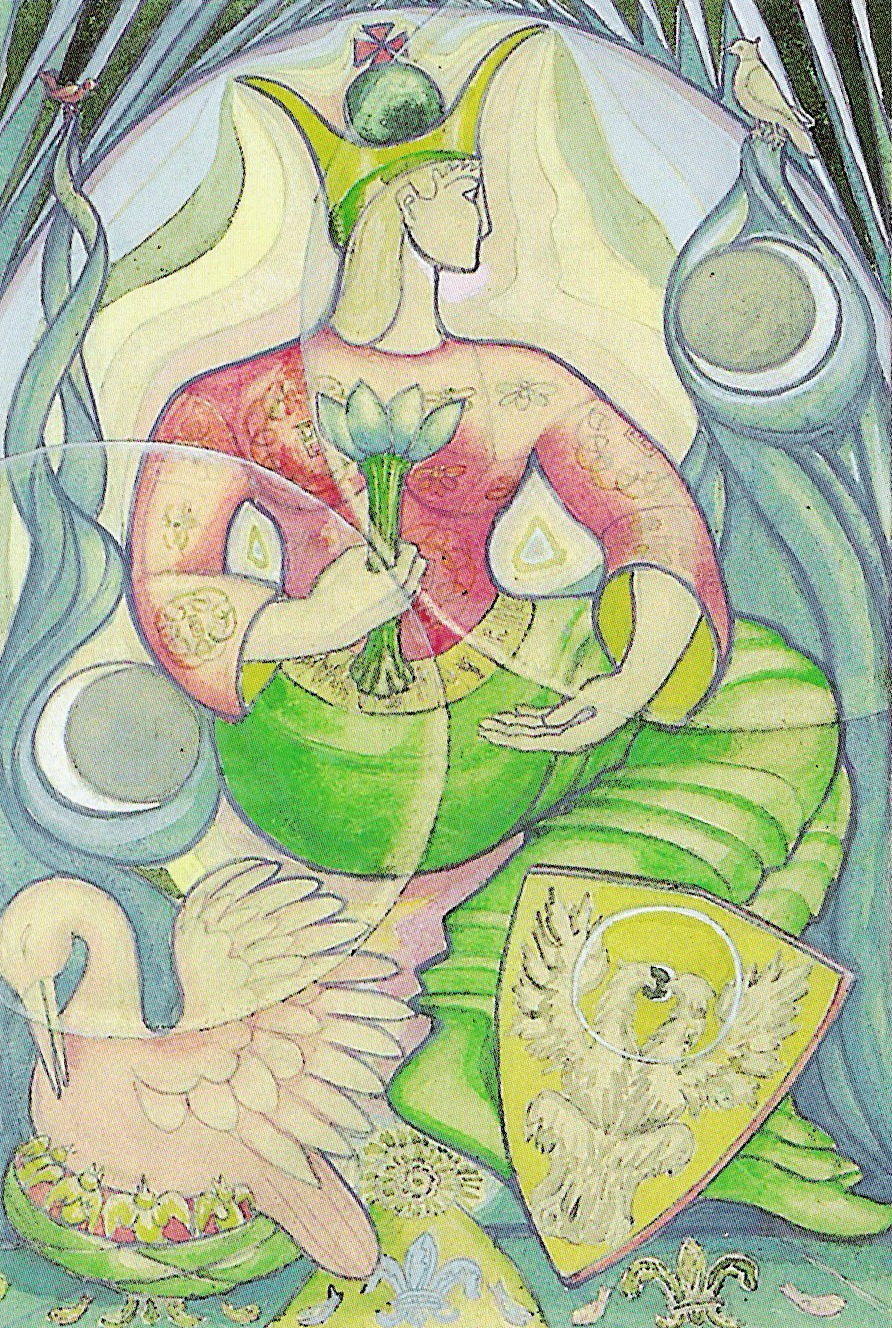The image is a richly detailed, two-dimensional painting with a blend of pastel and dramatic colors, exuding a contemporary Art Nouveau style with medieval influences. The central figure is a mermaid in a profile view facing right. The mermaid has long, flowing hair and a face that shares the same pale yellow hue as her hair. On her head sits a distinct hat featuring stems extending horizontally, topped with a green ball and a red cross.

Her attire is a tight-fitting suit that is predominantly red on her chest, with yellow extending along the arms, adorned with floral patterns. One of her arms is curled next to her stomach, clutching a white lotus flower, while the other arm is curved underneath her. Her mermaid tail starts from her waist, extending down to the left and then curving backward towards the bottom, colored in shades of green with subtle white highlights.

Among the surrounding elements, there's a yellow shield decorated with an open-winged bird located near where her feet would be, giving a medieval crest-like appearance. Adjacent to the shield, a white duck or swan with its head tucked down appears to be sleeping. Tiny birds are also scattered across the image, including a small red bird in the top left corner and a small yellow bird in the top right.

The background features additional symbolic elements, such as two half-moons flanking the mermaid, and a recurring three-leaf symbol present at the bottom, hinting at possible religious or symbolic significance. Despite the medieval stylistic techniques, the painting's use of bright and pastel colors lends it a modern, illustrative quality.